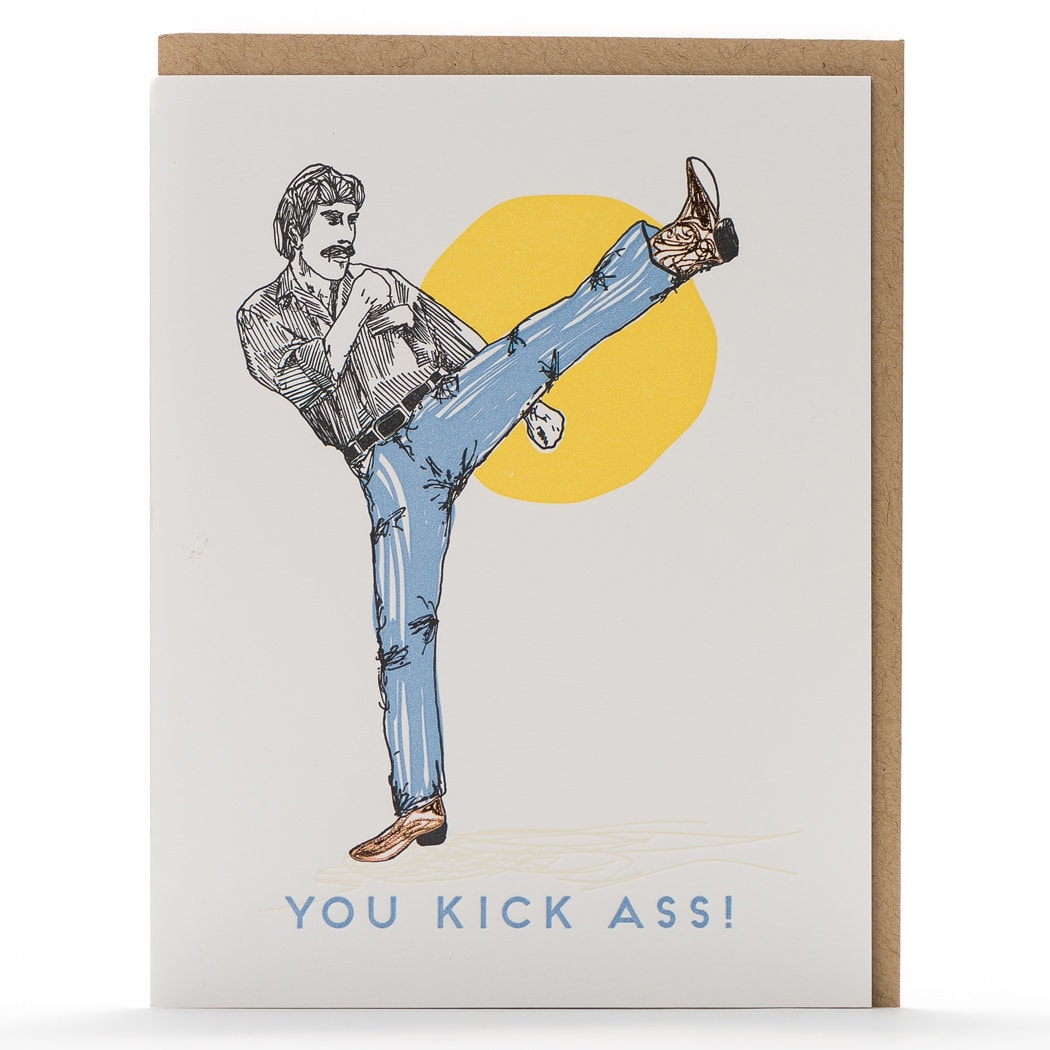This image resembles an old-school hand-drawn cartoon poster on white paper, bordered by a brown, recycled cardboard color, suggesting it might be a card with the envelope showing. At the center is a brightly painted yellow circle, symbolizing the sun. In front of the sun, a caricature of a man is depicted in an active, high-kicking pose. The man, drawn with thin black lines, sports long hair down to his ears, a mustache, and 1970s fashion. He wears blue jeans, a black belt, brown cowboy boots, and a black shirt adorned with thin white stripes and an unbuttoned collar. His left leg is thrust high into the air at a 45-degree angle, indicating a dynamic kick, while his left hand is positioned behind the raised leg. His right fist is clenched near his chin, emphasizing the action. The man's skin is white, and below him, in bold blue text, the words "You Kick Ass!" are prominently displayed.